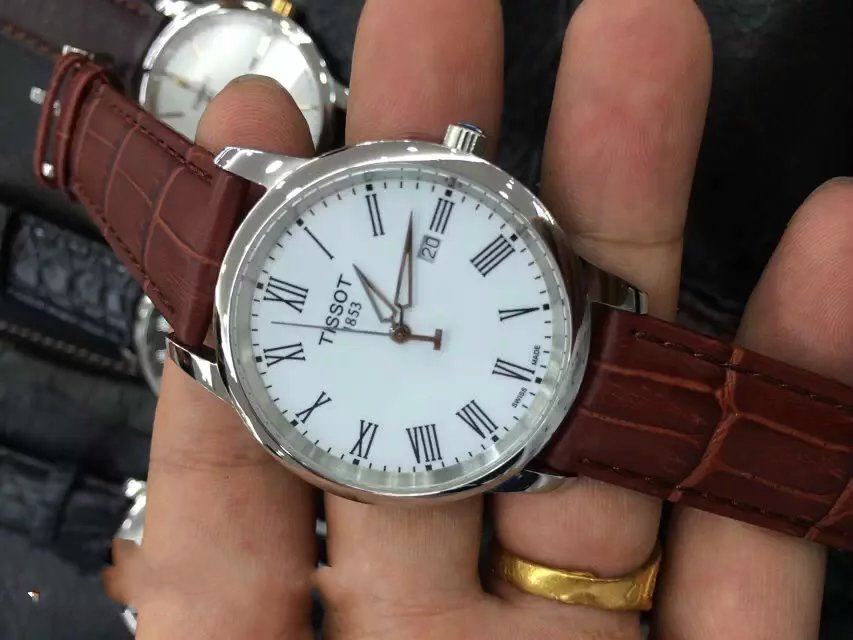A pale Caucasian hand is prominently featured, holding a round wristwatch. The hand, adorned with a gold ring at the base of the ring finger, displays an unusual glitch near one of the fingers, suggesting possible digital editing or AI generation. The watch boasts a silver back and dial, complemented by black Roman numerals for the numbers. The brand, "Tissot 1853," is clearly visible in the center of the watch face. The strap of the watch evokes a faux alligator texture and is a rich brown color, adding an element of sophistication to the image.